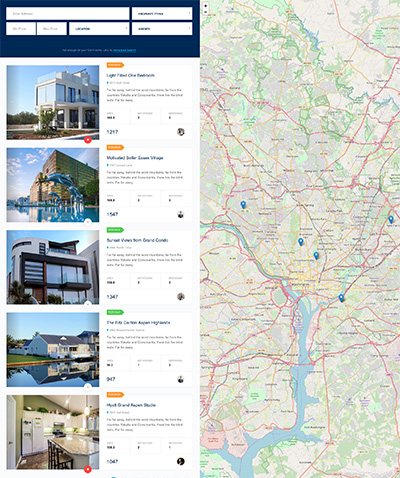The image captures a digital search session on a mobile device or computer screen, focusing on real estate properties. The interface is divided into two main sections: on the left side, there is a vertical list of property descriptions, accompanied by thumbnail images of each location. Above this list is a blue rectangular field with smaller white input areas, possibly for filtering search criteria. 

The property section showcases five different real estate options, though it is unclear whether they are for sale or rent due to the blurriness of the text. Additionally, three of these listings feature orange arrows beside them, while the remaining two have green arrows, likely indicating some form of interactive element or status indicator.

On the right side of the screen, there is a detailed map displaying a waterway towards the bottom and numerous red lines crisscrossing the area, symbolizing roads. Five pinpoints are marked on the map, corresponding to the locations of the properties listed on the left. The map provides a geographic context to the real estate listings, allowing the user to visualize where each property is located.